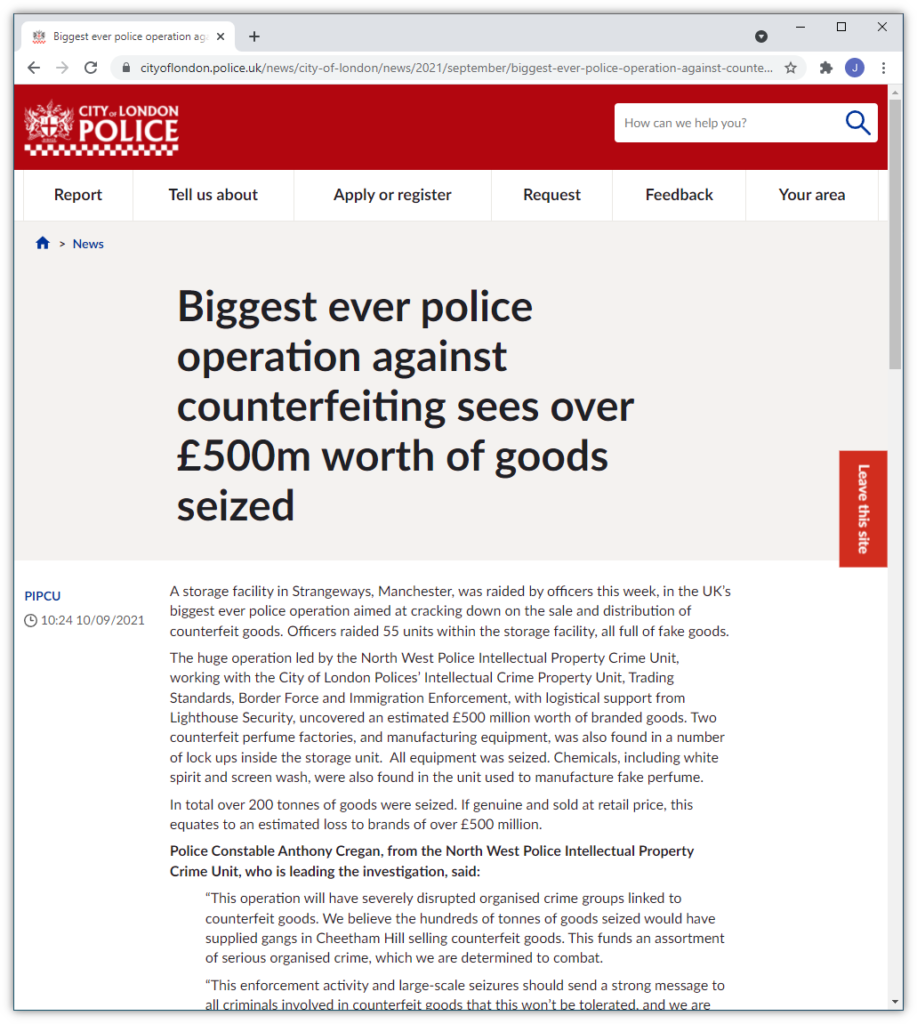**Screenshot of City of London Police Website Detailing Major Counterfeiting Operation**

In this screenshot of the City of London Police website, the browser is displaying a lengthy URL in the address bar. The site, cityoflondon.police.uk, features a prominent red header with the official City of London Police logo, which includes a distinguished crest with a shield and a red cross, bordered by a checkered pattern underneath both the badge emblem and the text.

At the top right of the page is a search field marked by the placeholder "How can we help you?" Flanking this are various menu options including "Report," "Tell us About," "Apply or Register," "Request Feedback," and "In Your Area." These options provide users with multiple ways to interact with and seek assistance from the police force.

Central to the page under the "News" section is a bold headline reading, "Biggest Ever Police Operation Against Counterfeiting." The subheadline details the magnitude of the operation, noting that over £500 million worth of counterfeit goods were seized. Below this headline is a substantial article beginning with the information: "A storage facility in Strangeways, Manchester was raided by officers this week," followed by four to five paragraphs extending off the bottom of the visible portion of the screenshot.

To the left side of the article, there is a timestamp that reads "PIPCU 10-24 on 10-09-2021," indicating the involvement of the Police Intellectual Property Crime Unit (PIPCU) and providing the date and time of the report. On the right side, an orange button labeled "Leave this site" is displayed vertically, offering users a quick exit from the page if needed.

Overall, the screenshot captures a detailed and serious announcement from the City of London Police regarding their largest-ever effort to combat counterfeiting activities.